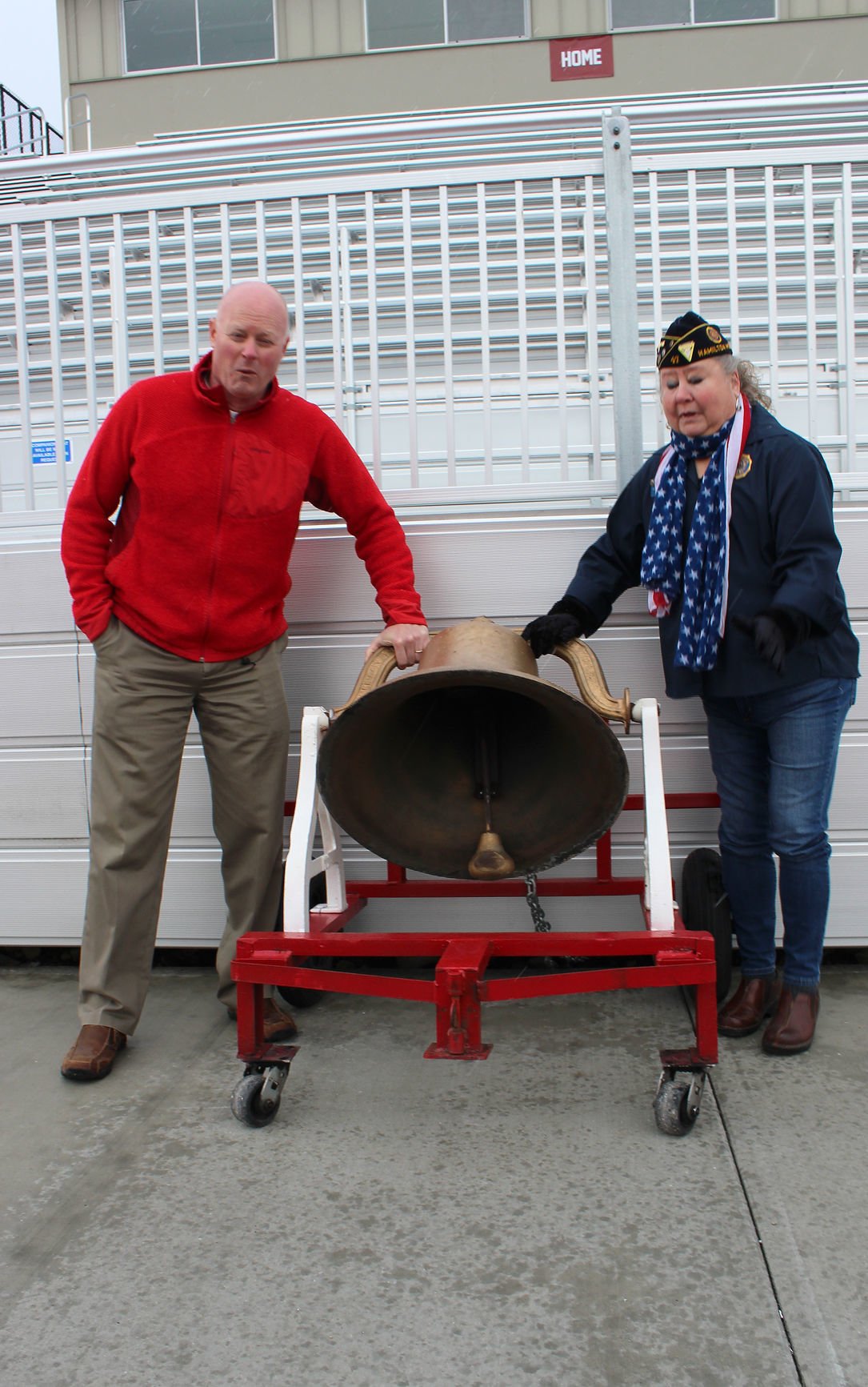The photograph captures a poignant outdoor scene featuring two individuals engaged in ringing a large brass bell mounted on a red and white metal frame with black caster wheels. The sky above is gray, indicating impending rain, with wet droplet marks scattered across the flat concrete surface below. On the left, a bald man dressed in tan-colored dress pants and brown leather shoes with black bottoms can be seen; he wears a red fleece jacket zipped up nearly to the collar. He uses his left hand to pull the bell backward. On the right, a woman with gray hair dons a navy blue jacket, blue jeans, and brown shoes. She wears an American flag scarf around her neck and a dark military garrison cap adorned with pins. Together, the man and woman work in tandem to ring the bell. They stand in front of a structure featuring a white-paneled wall and, further back, a stadium stand or press box with a red "HOME" sign in white letters.